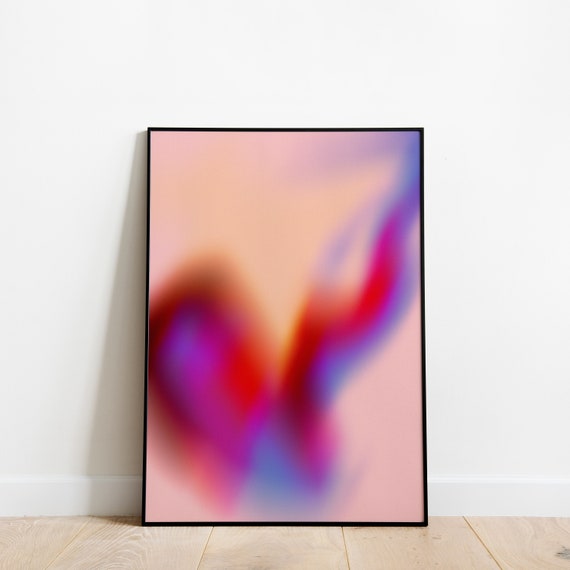The photograph depicts a painting leaning against a white wall, which includes a white baseboard, on a light-colored, wide plank hardwood floor. The painting is contained within a thin black frame. The artwork itself is abstract and features warm, wispy colors with a peachy-pink or golden pinkish background. Across the canvas, blurred swirls and smears of sunset reds, purples, and blues stretch from the lower half to the top of the image. The indistinct, diffuse forms in the painting seem to represent abstract shapes that each viewer might interpret differently.